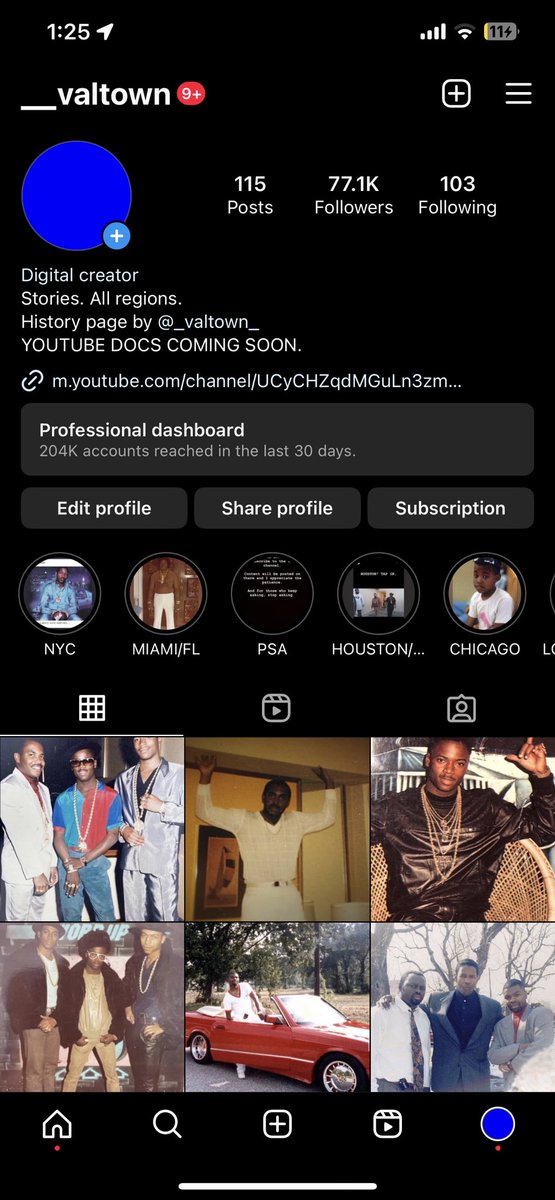The screenshot captures a mobile display of an Instagram profile, specifically focused on the account @underscoreValtown. In the top left corner, the time is indicated as 1:25 PM, accompanied by a location icon. The top right corner shows the Wi-Fi and cellular strength indicators along with a battery icon displaying 11% and a lightning bolt, suggesting the device is currently charging.

The profile header features a solid blue profile picture and the account statistics, which include 115 posts, 77.1K followers, and 103 following. Below the account name, the bio reads: "Digital creator, stories, all regions. History page by @underscoreValtown_YouTube docs coming soon," followed by a YouTube channel link.

The profile has a "Professional Dashboard" reporting that 204,000 accounts were reached in the last 30 days. Options for "Edit Profile," "Share Profile," and "Subscription" are also available. Just beneath these options, several circular icons suggest highlighted stories. The lower part of the screen displays a grid of six photos, each styled with a vintage aesthetic.